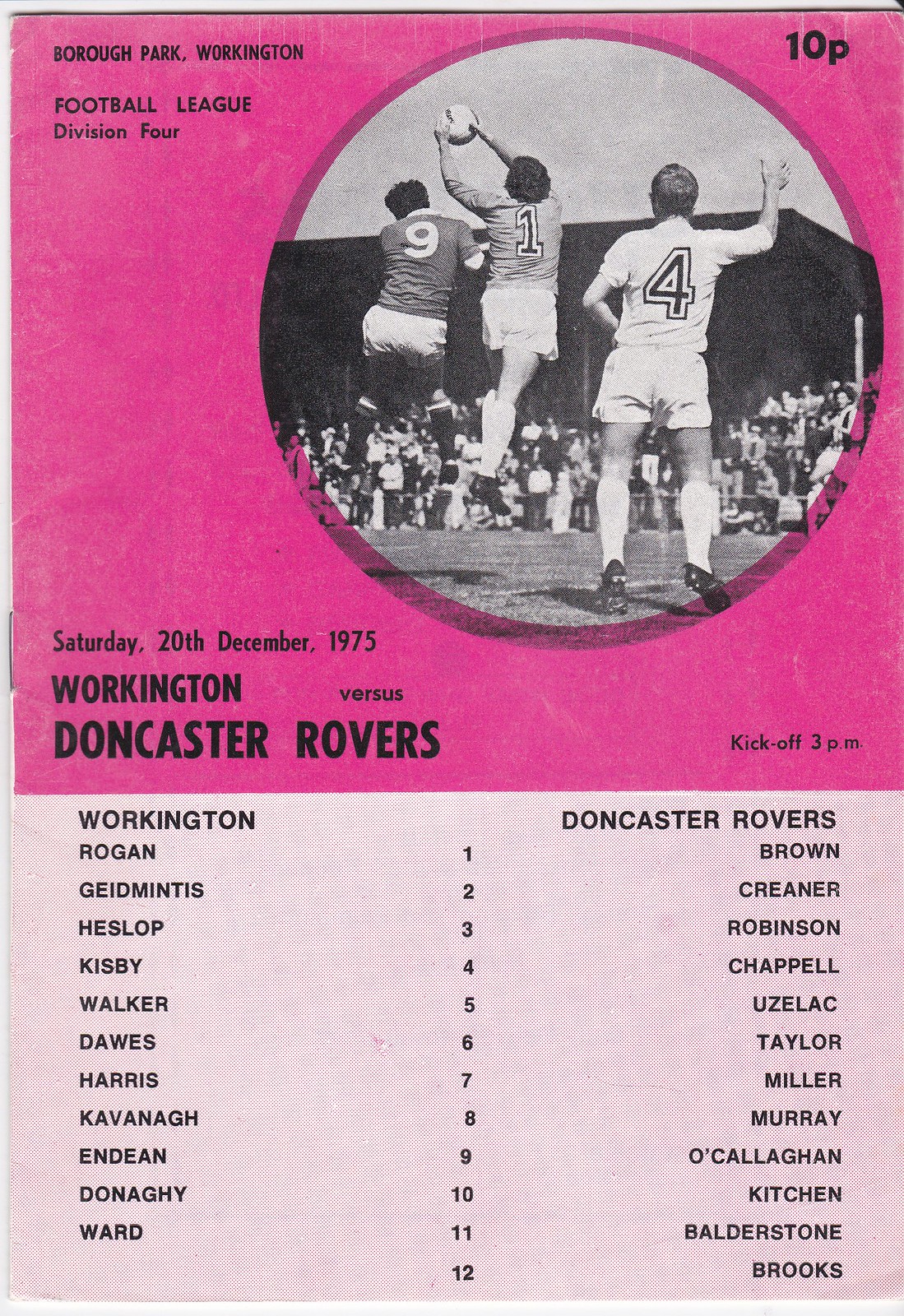This image is of a vintage football program with a two-tone design: pink at the top and white at the bottom. In the upper left corner, the text reads "Borough Park, Workington," followed by "Football League Division 4." The upper right corner displays the price, "10-P." Central to the layout, there's a large circular black-and-white photograph capturing an action-filled moment from a soccer match, featuring three players. One player, wearing the number 1 jersey, is airborne, clutching the ball, while the other two, with numbers 9 and 4, are engaged around him. The image background reveals the stadium, the audience, stands, and the sky. Below this photo, still within the pink section, the date "Saturday, 20th December 1975," the matchup "Workington vs. Doncaster Rovers," and "Kickoff, 3 p.m." are detailed.

Transitioning to the white section at the bottom, the left side lists the Workington team members: Rogan, Edmunds, Heslop, Kisby, Walker, Dawes, Harris, Kavanagh, Enden, Donaghy, and Ward. The right side lists the Doncaster Rovers players: Brown, Craner, Robinson, Chappell, Goselec, Taylor, Miller, Murray, O'Callaghan, Kitchen, Belterstone, and Brooks. A distinctive detail is a staple visible in the middle left, holding the program together. The overall effect is one of a meticulously organized and nostalgically preserved football match program.